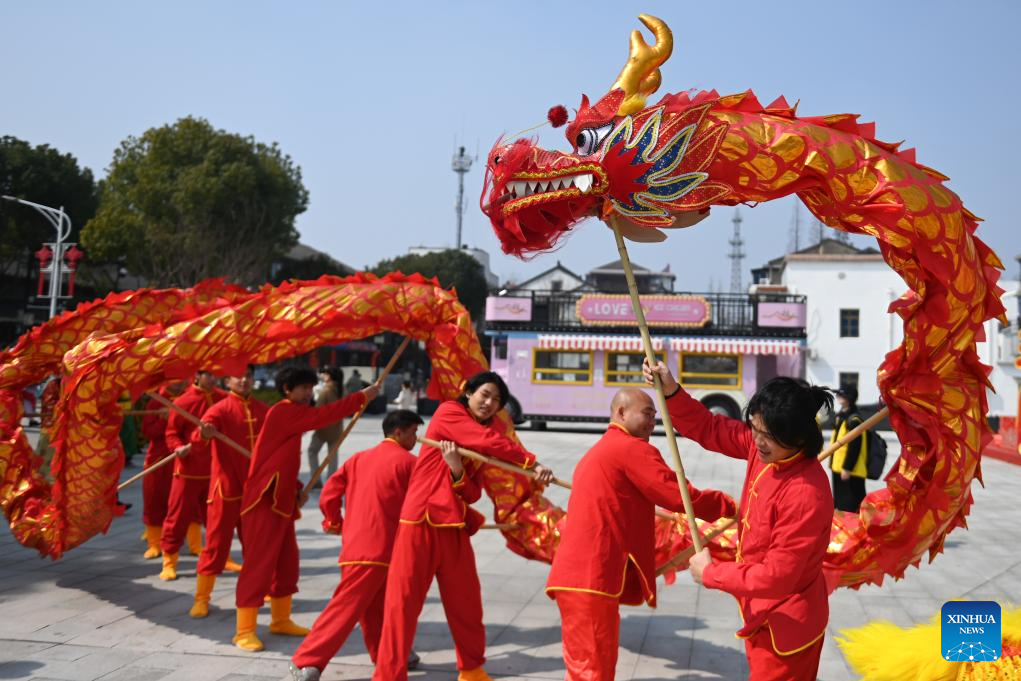This photograph captures a vibrant Chinese New Year parade featuring a life-size red serpent-like dragon puppet with golden horns and white teeth, maneuvered by a row of eight men dressed in traditional Chinese attire. Each man wears a red long-sleeve shirt and matching red pants with gold trim, along with distinctive yellow boots. The dragon, held aloft by sticks, appears to be floating and curling through the air as the performers skillfully control its movements. The scene is set against a backdrop of a clear blue sky with scattered trees, a white building, and a pink and white food stand with yellow-trimmed windows. In the lower right corner, the text "XINHUA News" is visible in white letters within a blue box, adding to the event's celebratory atmosphere.